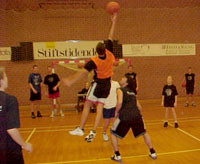In this photograph, a group of students are engaged in a lively game of basketball, likely part of a gym class given the mix of ages among the participants. The setting appears to be a school gymnasium, characterized by its tan-colored hardwood floor and matching tan walls. White signs with black text are mounted on the walls, providing necessary information or instructions typically found in school settings. 

In the background, a red and white striped goal, resembling a soccer net, adds to the multi-purpose nature of the gym. Center stage, a student in black shorts and a vibrant yellow shirt leaps into the air, arm fully extended, as he reaches for the basketball. Surrounding him are three to four other students, mostly dressed in black shirts and shorts, with one child standing out in red shorts. The small size of the image makes finer details difficult to discern, but the energy and dynamism of the scene are clearly evident.